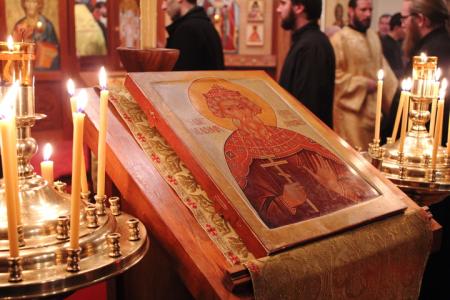The image depicts a solemn religious ceremony, likely set in a Russian or Greek Orthodox church. At the center of the scene is a revered icon resting on a pedestal adorned with an embroidered cloth. The icon features a religious figure dressed in rich robes and a distinctive red hat, holding a unique cross with three arms in the right hand and presenting an open left palm. On either side of the icon, tall candle holders illuminate the sacred space, casting a gentle glow. In the background, a group of men clad in religious attire, some in yellowish-white sacramental robes, are engaged in conversation and viewing other religious artworks hanging on the walls. The atmosphere is deeply reverent, with the light from the candles enhancing the spiritual ambiance of the ceremony.